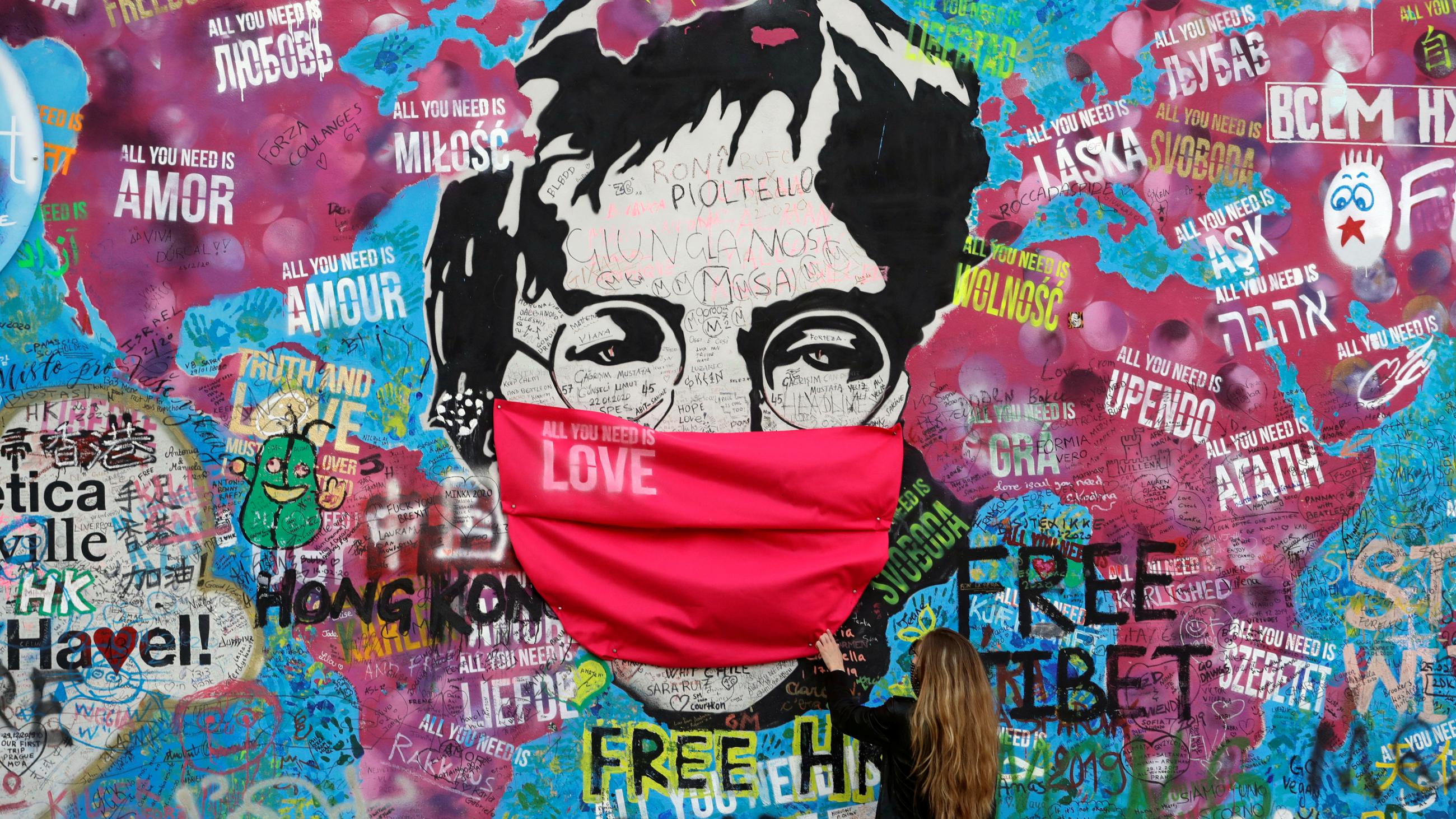This image depicts a vibrant outdoor mural featuring a multitude of colors and elements. Dominating the mural is a large, black-and-white depiction of what appears to be John Lennon, his face adorned with glasses and partly obscured by a protruding, red cloth face mask that declares "All You Need Is Love." A real-life woman stands in front of the mural, interacting with the mask.

On the left side of the mural, the outlines of North and South America are rendered in a pinkish hue, juxtaposed against the bright blue representation of oceans. To the right of the central figure, the outlines of Africa, Europe, and Russia continue the pinkish color scheme. Scattered across the mural are various words and slogans, including "Free Tibet" and "Hong Kong," as well as translations of "All You Need Is Love" in multiple languages. The mural integrates these diverse elements into a harmonious, multicolored collage that conveys a message of unity and love.